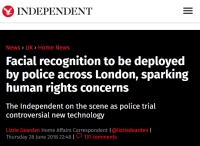On a black background, there is a prominent red circle featuring a white eagle in the center. To the right of this emblem, there is a gray hamburger icon. The image includes text, though much of it is too small to read clearly. However, the text in the foreground reads: "Facial recognition to be deployed by police across London, sparking human rights concerns." Below this, in smaller text: "Independent on the scene as police trial controversial new technology." Additionally, there are two words in red, and three words in white, but they are not legible. The date mentioned includes "Thursday" and appears to be around the late 20s of June, possibly June 28 or 29.